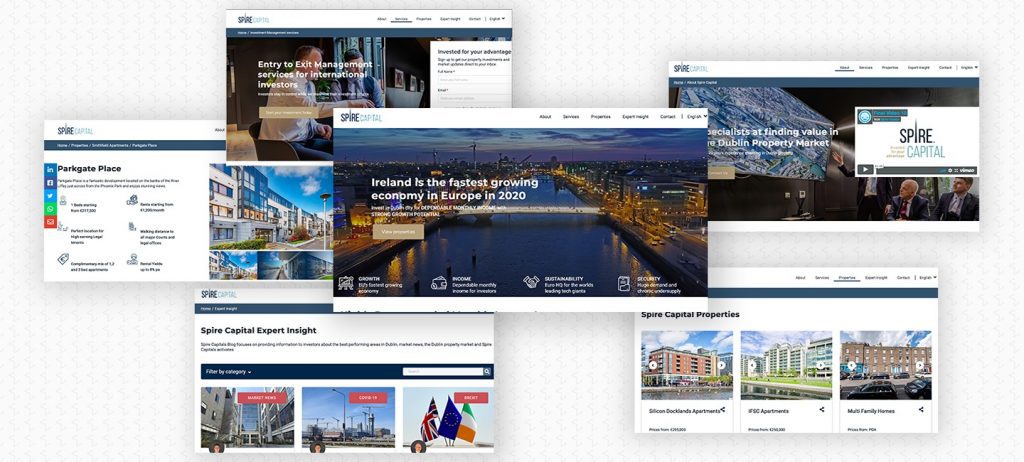This image features a collection of six thumbnail screenshots depicting various websites, arranged in two rows against a white gradient background. The first screenshot, located at the top left, showcases an opt-in form with two men and a headline stating "Ireland is the fastest-growing economy in Europe in 2020," accompanied by an image of Ireland. Below this are computer-generated images of buildings.

To the right of the initial screenshot, additional thumbnails are displayed side by side. The second thumbnail includes an Irish flag, a British flag, and a third blue flag, possibly representative of various nations or entities. The final screenshot in the sequence features images of three different buildings, all branded under the name "Spire Capital Properties." Each building includes the "Spire Capital Properties" label, indicating they belong to the same real estate company.